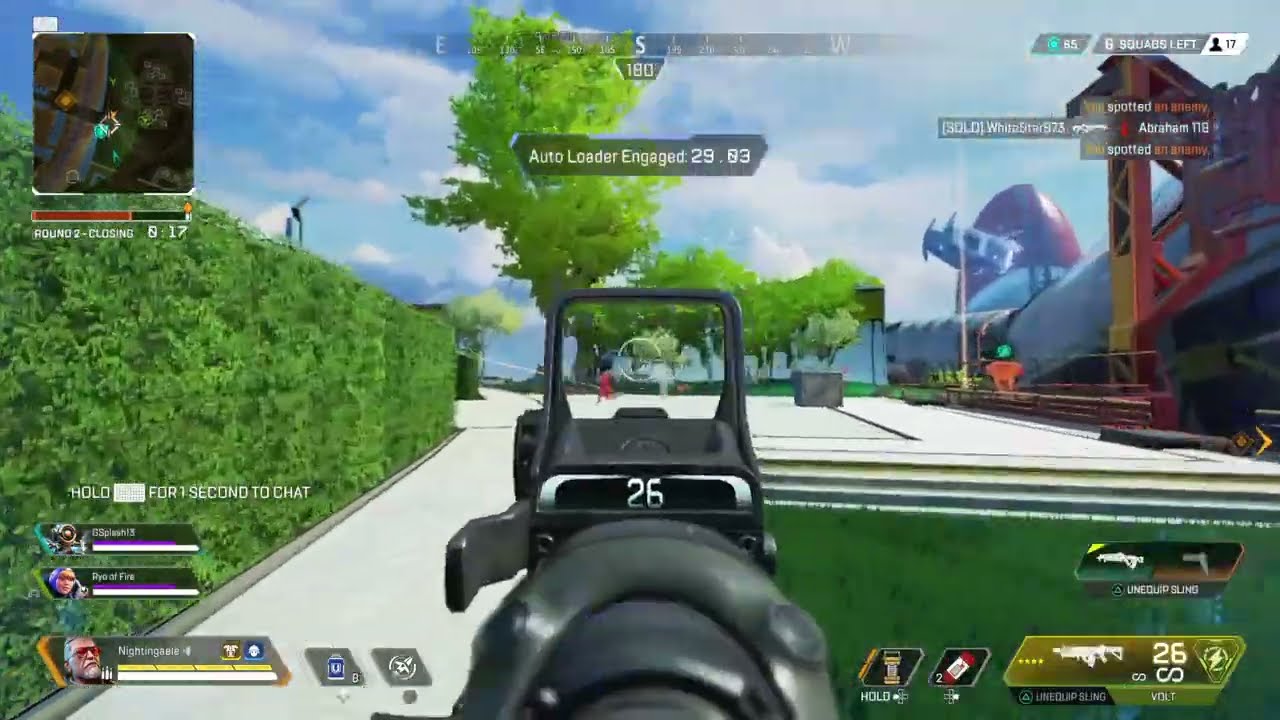In this first-person perspective image from a video game, the player is viewing the scene down the barrel of a black rifle with a digital ammo count display showing 26 bullets. The rifle has a square sight attached on top. The environment features a white ground with a rectangular wall of green hedges on the left, trees in the background, and steps leading up to a building structure supported by red metal bars on the right. An opposing character, dressed in red pants and a black hoodie, is visible off in the distance, running through the area.

The game's UI is prominently displayed: at the bottom left, icons of three teammates are shown, including the main character "19EggGale," "Ryo of Fire," and "O-Splash13," with blurred text above them. An orange bar indicates time progression for "round two," which is "closing in 17 seconds." The top left corner houses a mini-map, while the top of the screen features a compass pointing south (180 degrees). In the top right, the interface shows "65" health points, "six squads left," and "17 players remaining." There is a kill feed indicating "You spotted an enemy," and combat updates involving players "Solo Wimstar 573" and "Abraham 118."

Additionally, in the lower right, there’s an hourglass symbol and a red dynamite-shaped grenade icon next to the ammo count and an infinite symbol, suggesting unlimited ammunition. Above the gun’s ammo count, text reads "auto leader engaged" with a figure "29.03." The various UI elements and the detailed scene create an immersive and complex gaming interface.